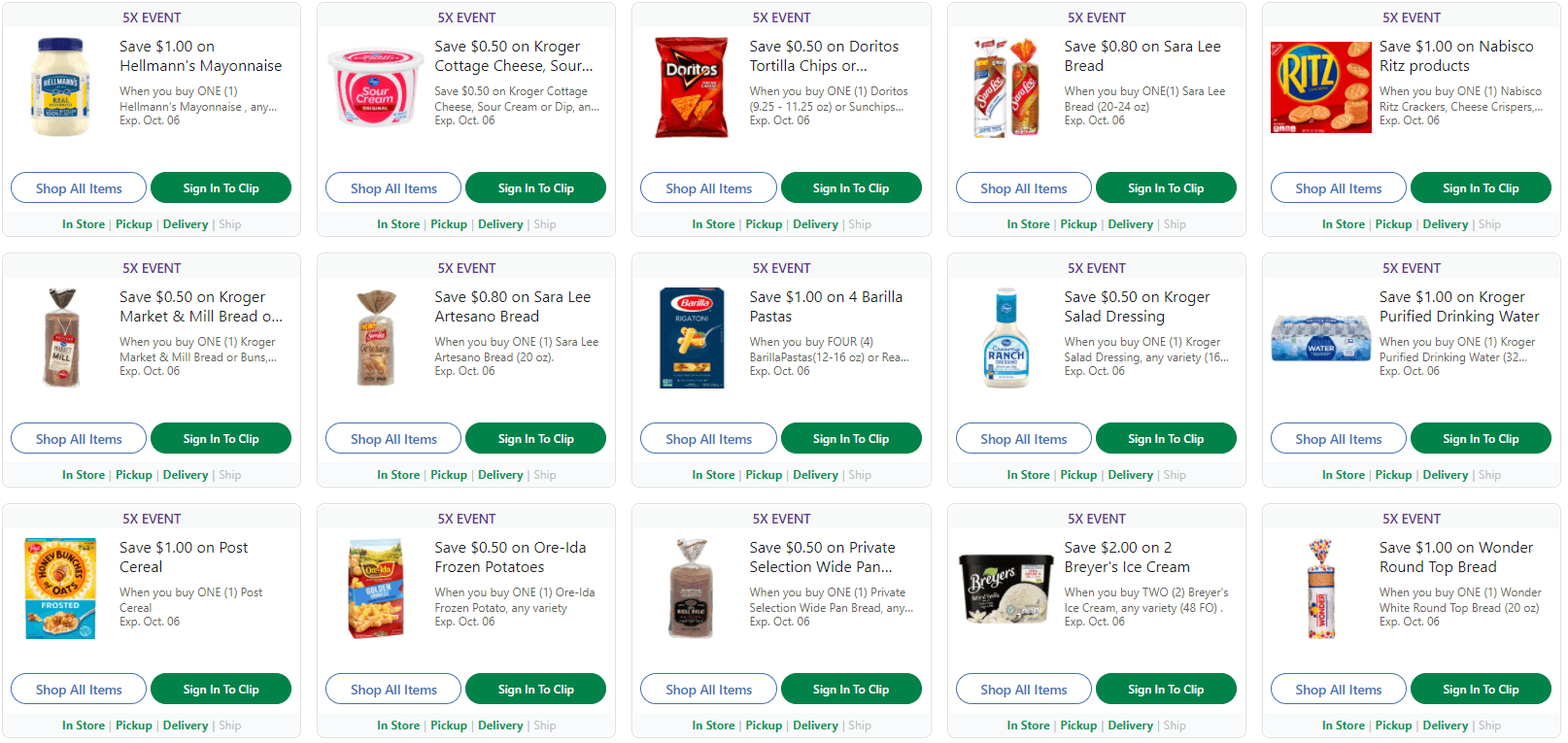This image depicts a section of an e-commerce website focused on food and beverage products. The layout reveals a grid of 15 items, organized into three rows with five products per row. Each product is displayed with a high-resolution color photograph and detailed information.

Across the top row, the products include Hellmann's mayonnaise, cottage cheese, Doritos chips, bread, and Ritz Crackers. The second row features another type of bread, additional bread variety, pasta, ranch dressing, and bottled water. The bottom row showcases cereal, possibly frozen potatoes, more bread, Dreyer's ice cream, and Wonder Bread.

Accompanying each product image is a label "SX EVENT," printed in all caps, followed by a statement indicating the savings ("SAVE X AMOUNT OF MONEY"). There is also very small text providing details on the conditions of the purchase, such as quantity or membership requirements. Below the text for each product, two capsule-shaped buttons are available: a white "SHOP ALL ITEMS" button on the left, and a green "SIGN IN TO CLIP" button on the right, facilitating a seamless shopping experience for users.